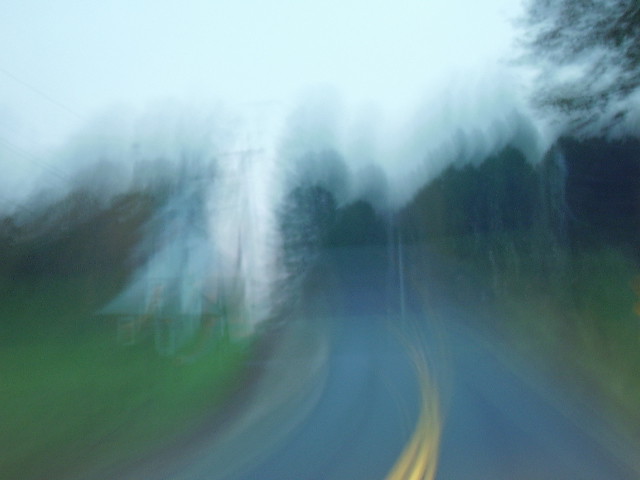The image depicts a very blurry road scene. The entire image lacks clarity, with the road in the center and the surroundings on both the left and right sides appearing indistinct. At the bottom center, a road with gray pavement is visible, marked by yellow lines that fade out shortly after entering the frame due to the blurriness. On the left side, the ground is green, indicating the presence of grass, which is also visible on the right side. Above the grass, a series of faded and blurry lights and colors create a mixed layer of white on the left, transitioning to light blue, and then to brown. In the background, there are vague outlines of trees, and above them, the sky appears in a bluish-white hue.